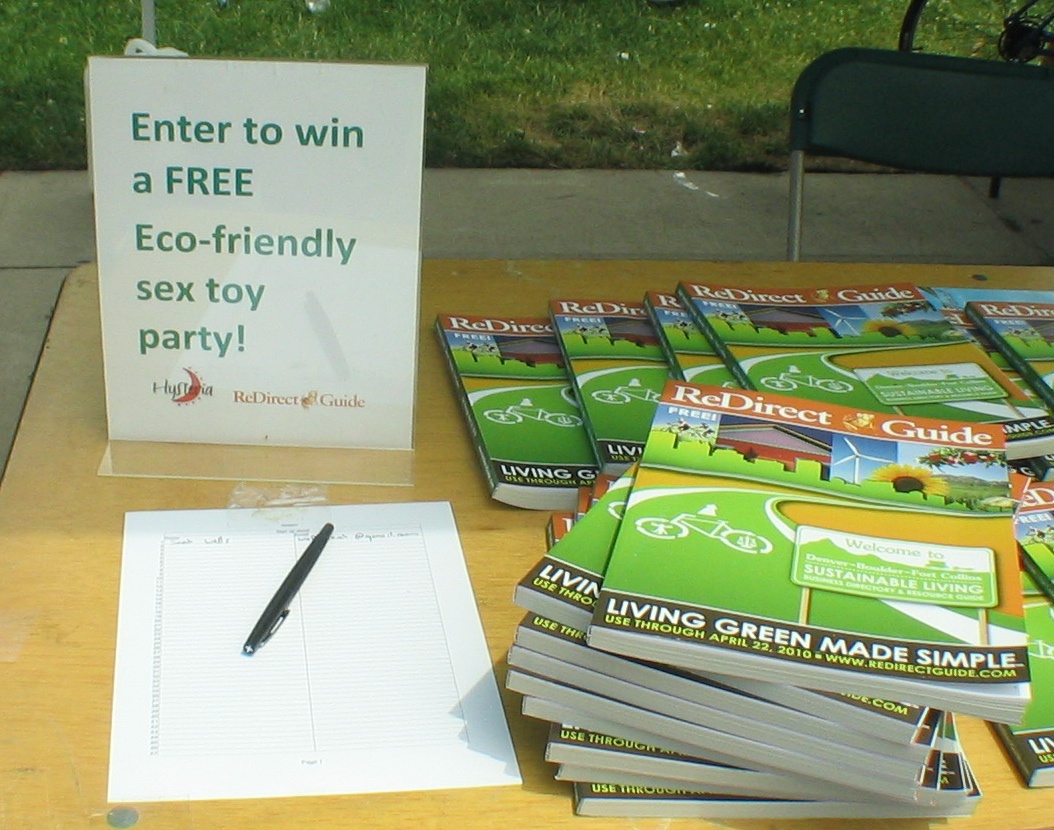A natural wood-colored table is set up, possibly for an outdoor event, featuring various informational materials and sign-up opportunities. Dominating the table are stacks of thick brochures titled "Redirect Guide: Living Green Made Simple," complete with covers depicting a bicycle and a pathway. Adjacent to these brochures, on the left side of the table, lies a sign-up sheet pinned down for people to leave their names. 

Above the sign-up sheet, encased in a transparent, double-sided plastic holder, is a prominent white sheet with green text proclaiming, "Enter to Win a Free Eco-Friendly Sex Toy Party." The bottom of this sheet displays two company logos, one notably featuring a red crescent moon paired with aligning dots. In front of the table, a fold-up chair awaits participants. This unusual combination of materials aims to promote an eco-friendly lifestyle while offering a quirky incentive for engagement.